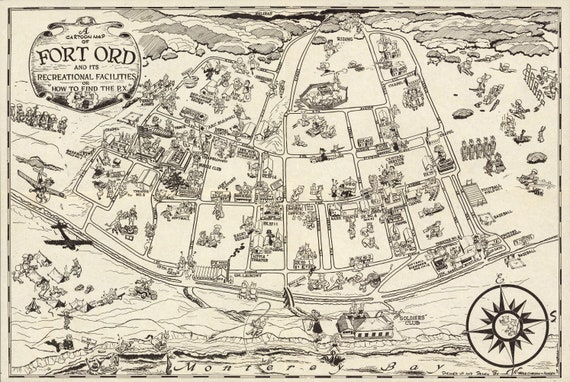The image is a scanned, hand-drawn map displaying an aerial view of an area labeled "Fort Ord and its Recreational Facilities" in the upper left corner. This cartoon-style map is primarily black and white with an off-white cream background. It illustrates various roads, buildings, and houses in a neighborhood. At the bottom right corner, there is a meticulously drawn compass featuring a star pattern and a globe in the center, standing out from the otherwise hand-drawn elements of the map.

In the lower portion of the map, "Monterey Bay" is labeled, indicating its geographic context. The map also includes various graphical elements such as clouds and airplanes in the sky, and on the right side, there is an illustration of people standing in formation, presumably participating in some type of training. The detailed and whimsical nature of the map suggests a mix of practical layout and artistic embellishments, providing a comprehensive overview of Fort Ord and its surroundings.